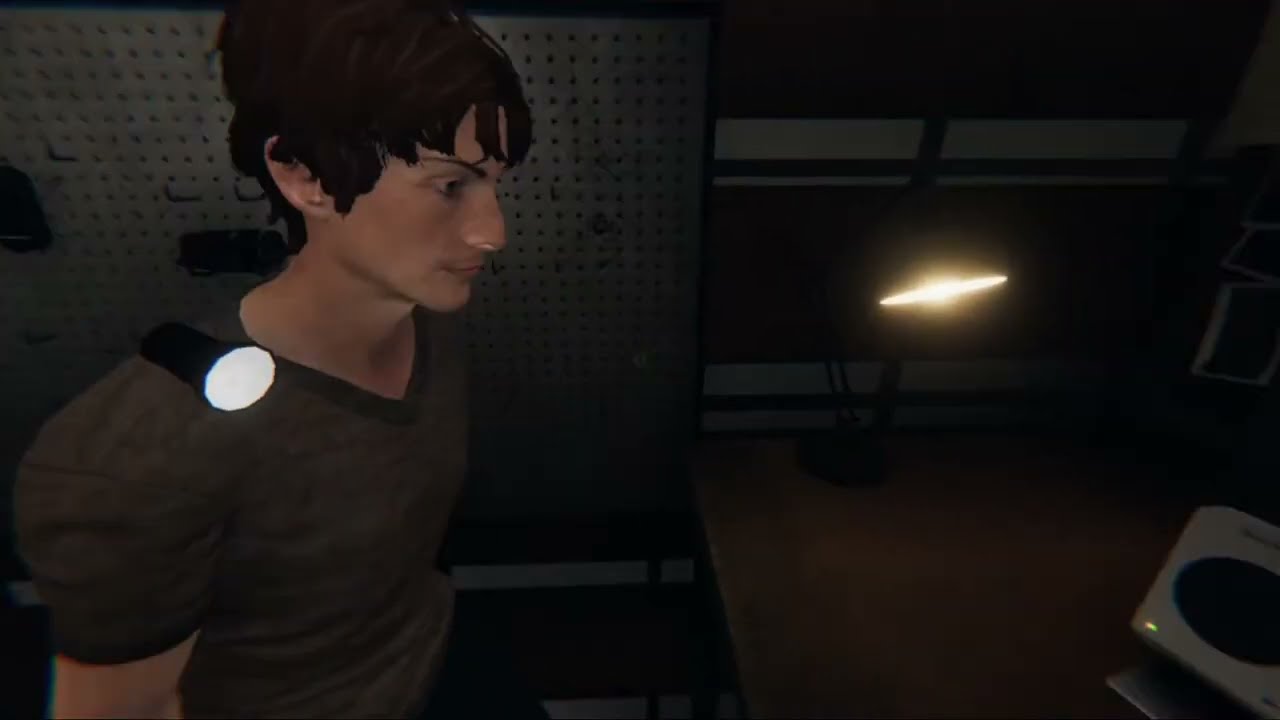The image appears to be from a video game, featuring a male character whose semi-realistic appearance still identifies him as a digital creation. The man, with his disheveled brown, shaggy hair and thin upward-angled eyebrows, sports a dark green or possibly brown v-neck t-shirt with short sleeves, revealing a bit of his arm. He has a flashlight clipped to his right shoulder, casting light on his white, Caucasian skin. His face, characterized by a biggish nose and intense expression, is the focal point, illuminated against the otherwise dimly lit scene.

The setting behind him resembles a workshop or a cluttered room. On the left side of the background, a large white pegboard with hooks is visible, housing a few items. To the right, the character is facing a brown workbench or table, on which sits a glowing black lamp emitting a yellowish light. A white machine, which might be a robot, is situated in the bottom right corner, and a poster or corkboard with holes hangs nearby. The scene is predominantly dark, making the illuminated elements and the character's focused demeanor stand out in the shadowy environment.